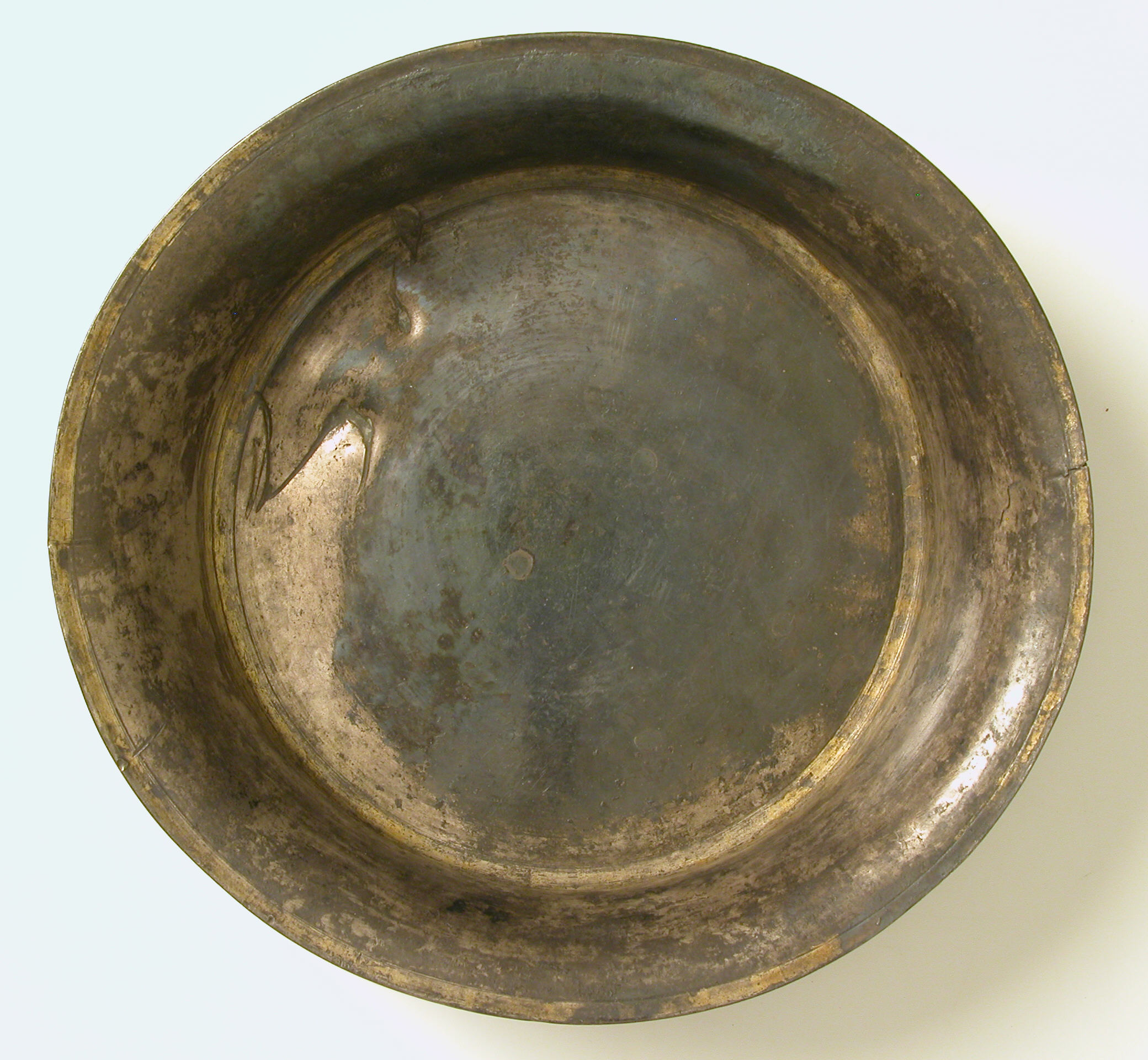The image features a very old, distressed metal plate, likely made from a material such as copper or iron, evident by its tarnished, brownish hues ranging from dark to light brown. The plate, covered in noticeable patina, displays discoloration, scratches, and grime, which suggests significant aging. Distinctive gold rims, now faded, once adorned both the outer and inner edges of the plate, adding a touch of elegance amidst the wear and tear. The middle of the plate is particularly dark and oxidized, with scratches and dings suggesting it has seen rough use, possibly even in a military context. Some light shines through areas where tarnish has worn off, revealing a metallic or bronze-like sheen. The plate sits on a light blue surface, which contrasts its aged, dingy appearance.